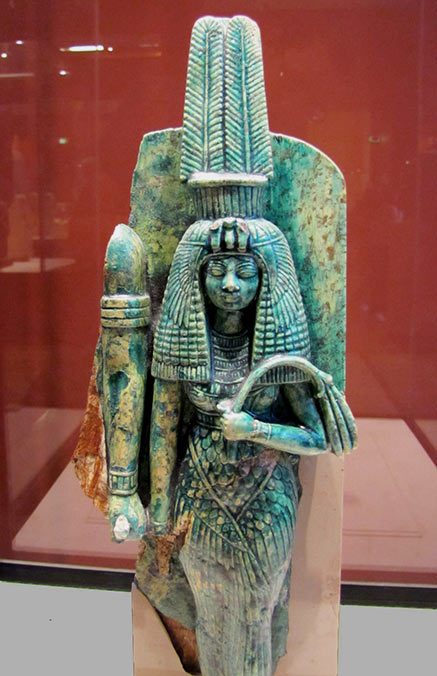The image features a close-up of an intricately carved historical statue, likely of an Egyptian woman, possibly dating back to ancient times. The statue appears to be displayed in a museum, encased behind glass with a red and pink base and a white backdrop for support. This Egyptian female figure is adorned in a ceremonial headdress, which is elaborate and seems to feature a cobra or bird motif with patterned wings above the forehead. Her eyes are closed, she's holding what seems to be a floppy-looking flower or a whip in her right hand. The dress she wears resembles dragon scales in its detailing, and the statue is made from a bluish-green stone with specks of white, dark brown, and black, potentially jade or turquoise. Behind her, there's a fragment of what appears to be an arm of another statue, possibly suggesting the remaining piece of a larger ensemble, like a depiction of a woman and her damaged husband statue beside her.